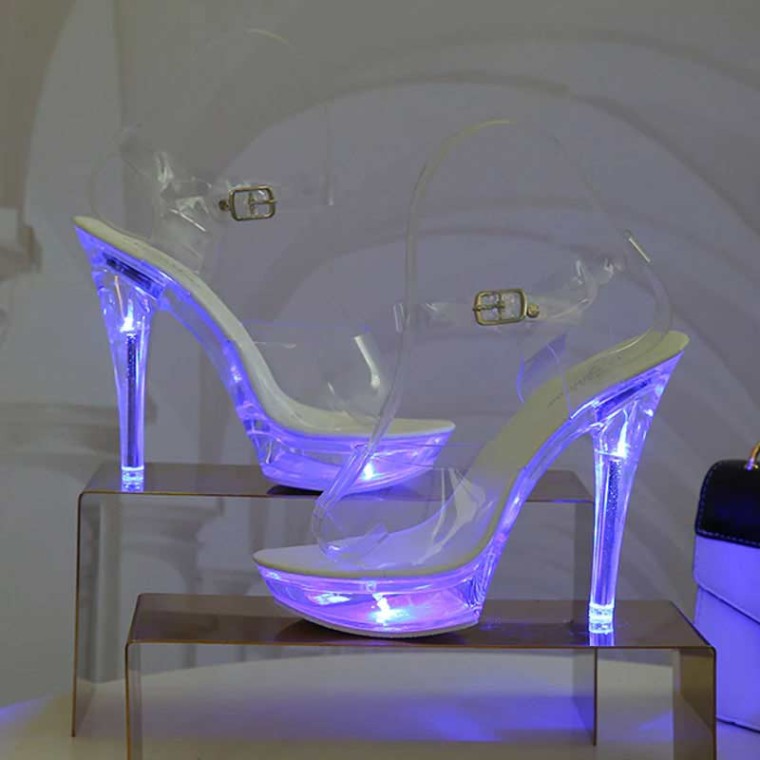The photograph shows a pair of high-heeled shoes, elegantly displayed on two acrylic risers against a light gray wall with dark gray shadow arcs. The risers are rectangular, the one in the front standing about an inch high and the one in the back about twice as tall, both approximately three inches wide. The shoes are made from a purplish-white plastic or acrylic that reflects light, giving them an electrifying glow, possibly enhanced by LEDs inside the soles. The shoe in the front faces left with its heel on the right, while the one in the back faces right with its heel on the left. Each shoe has clear plastic straps over the toes and around the ankles, secured with gold clasps. Transparent foot-shaped forms have been inserted to maintain the shape of the shoes, highlighting the clear straps that adorn the footwear.